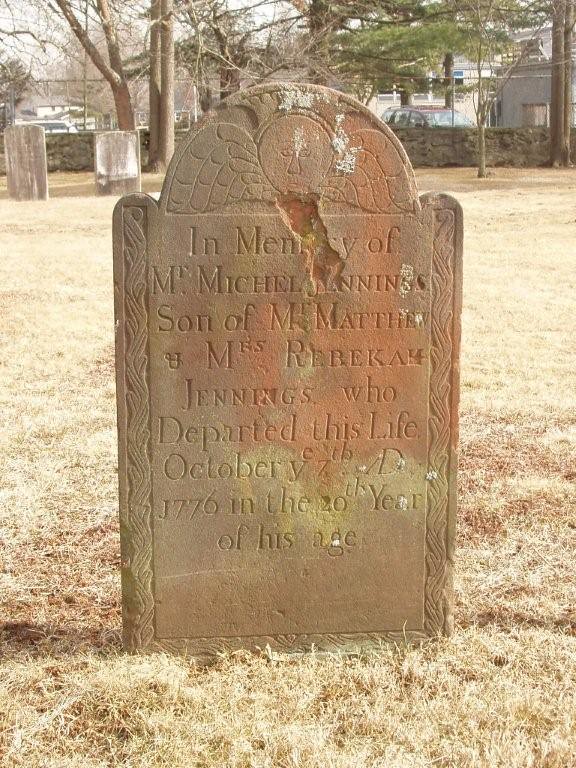This photograph, set in a cemetery during the likely winter months, captures a weathered tombstone surrounded by a vast expanse of greenish-yellow grass, indicative of the season. The background features sparse, nearly leafless trees, a few old-looking tombstones, and distant houses and cars, suggesting a less crowded graveyard. The focal point of the image is a cracked and aged gravestone, adorned with the faintly eerie visage of an angel at the top, complete with a face and wings. This gravestone bears the inscription: "In memory of Mr. Mitchell Jennings, son of Mr. Matthew and Mrs. Rebecca Jennings, who departed this life October 7th, 1776, in the 20th year of his age." The tombstone's surface is marred by white gunk and a significant piece missing from the front, further emphasizing its antiquity and historical significance.